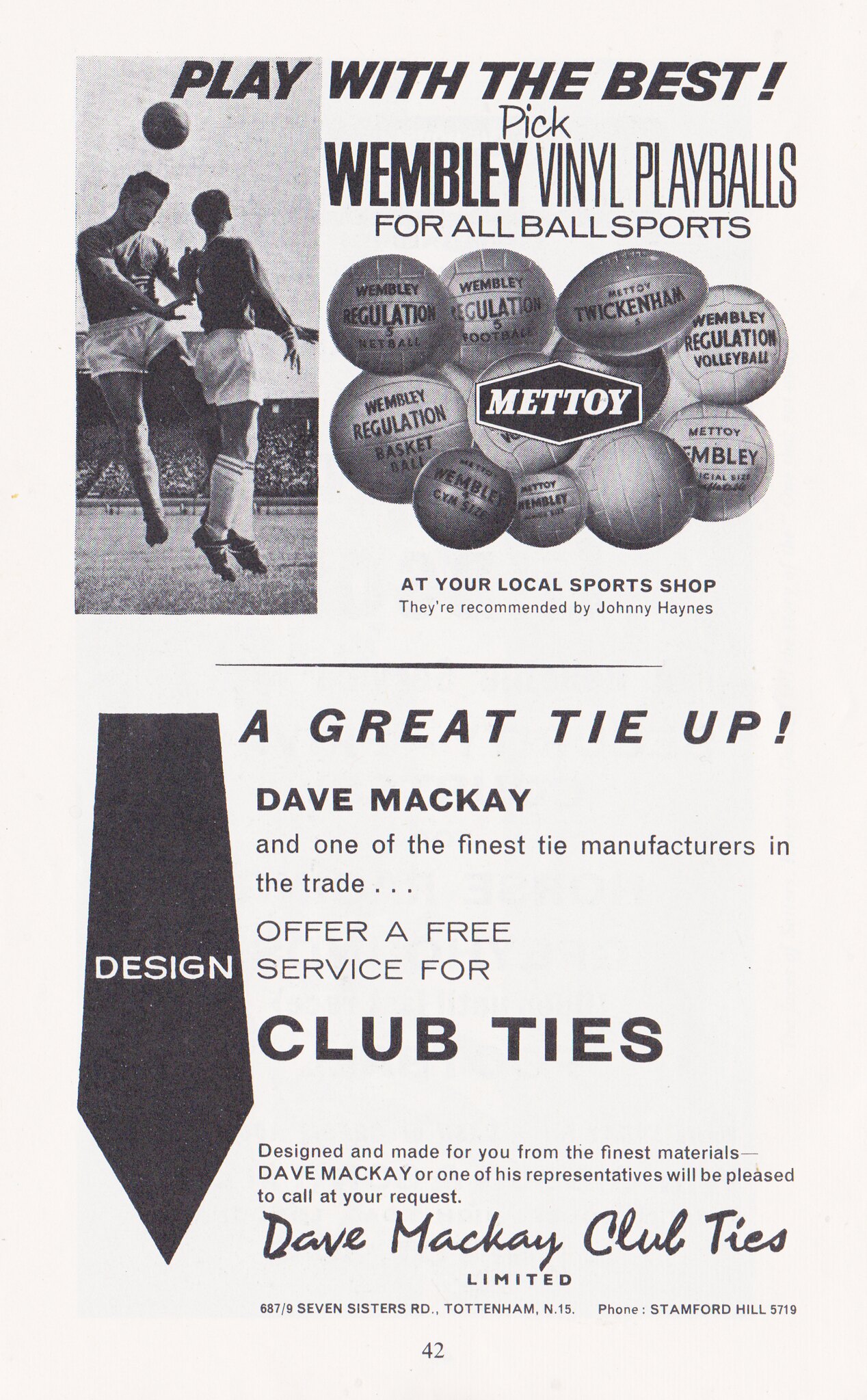The black-and-white image appears to be a scan from a magazine or program page, printed on plain, creamy white paper, primarily featuring advertisements. At the top, the bold black text states, "Play with the Best," followed by "Pick Wembley Vinyl Play Balls for All Ball Sports." To the left, a photo depicts two men in sports uniforms on a soccer field, one seemingly bouncing a ball off his head. Below this, various types of balls, including a football, basketball, volleyball, netball, rugby ball, and gym balls, are displayed with descriptions like "Wembley regulation volleyball” and “Wembley regulation netball.” The balls are associated with the logo "Mettoy" and are recommended by Johnny Haynes. The advertisement concludes with the statement, "Available at your local sports shop."

The bottom half of the page features another ad, introduced by the text "A Great Tie-Up." It showcases Dave McKay, described as "one of the finest tie manufacturers in the trade," offering a free design service for custom club ties made from premium materials. An oblong black tie with "design" written in white letters is pictured next to the text. The advertisement promises that Dave McKay or a representative would be pleased to arrange a meeting upon request. The company’s name, "Dave McKay Club Ties Limited," is written in a handwritten-style font, with the address "687-97 Sisters Road, Tottenham, N15," and a contact number "Phone: Stanford Hill 5719." The page is marked as page 42.